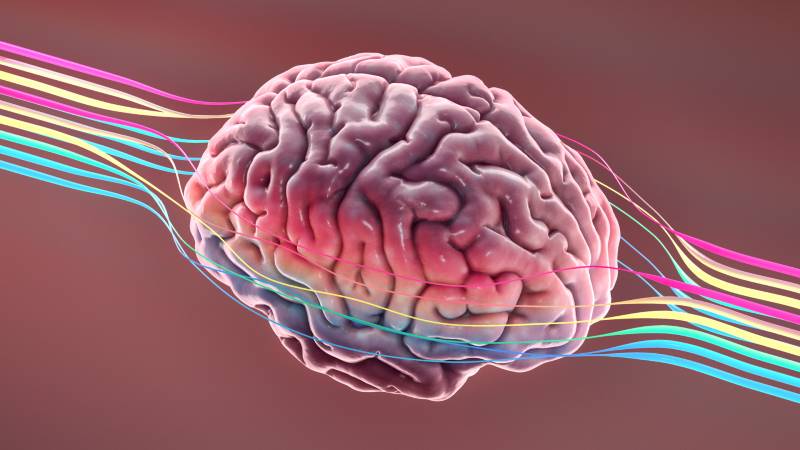The image depicts a detailed, computer-generated representation of a human brain, complete with intricate ridges and grooves typical of a real brain. Surrounding and weaving through the brain are ribbon-like electrical fields in vibrant colors, including pink, yellow, and blue. These colorful ribbons, which may represent electrical activity or wavelengths, appear to move dynamically around the brain, extending from the front to the back and creating a visually striking effect, reminiscent of a rainbow. The composition sits against a light purple or beige background, enhancing the vividness of the brain and the swirling, multicolored ribbons.